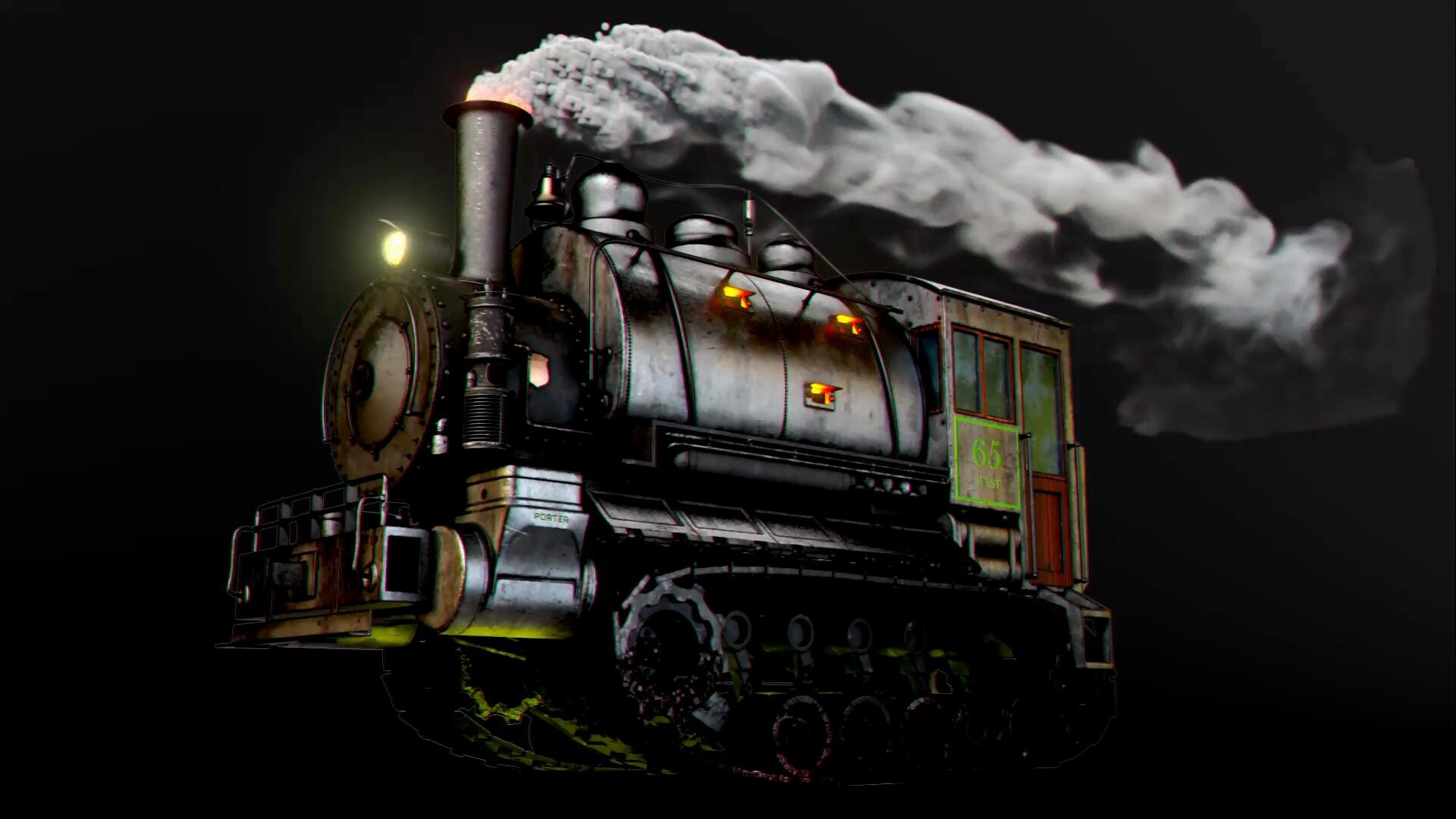In the center of this very dark image, set against a completely black background, stands a detailed and stylistic depiction of an old steam locomotive. The imposing black body of the train reflects light, accentuating its metallic features. Front and center, a bright yellow headlight pierces through the darkness. The locomotive is spewing large billows of grayish-white smoke from its prominent black smokestack. The train rests on black tracks, with a notable contrast provided by a more silver, cylindrical area near the top. To the back, there is a minor rusty section, and to the right of the train's front, a light green box bearing the number "65" is visible, likely indicating the engine number. The entire scene has a digitally rendered, almost cartoon-like quality that enhances its stylistic charm.